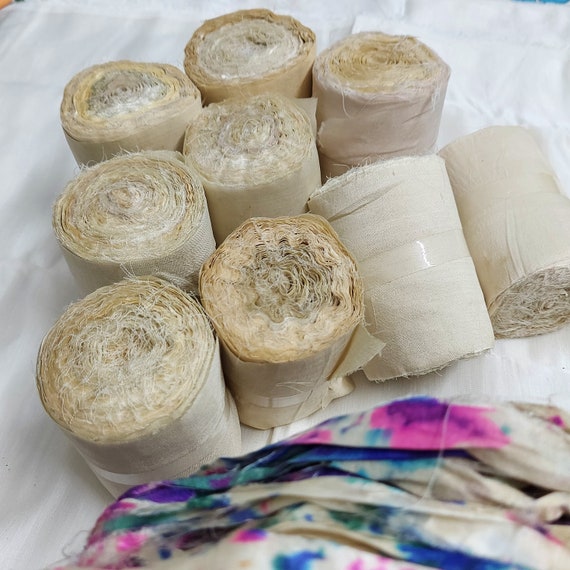The image features nine tightly coiled rolls of a beige to tan cloth material, resembling gauze or unprocessed linen with rough, frayed edges. These rolls, each approximately four to five inches tall, are secured in their cylindrical shape with bands of clear plastic or scotch tape around the center to prevent them from unrolling. Seven of the rolls are standing upright on a white sheet, while the two in the bottom right corner are tipped over on their sides. The cloth appears aged, with some parts displaying browning or warping, suggesting it may have absorbed moisture over time. The background includes a partially visible floral-patterned fabric with purple and blue flowers, providing a contrast to the simplicity of the coiled cloth rolls.